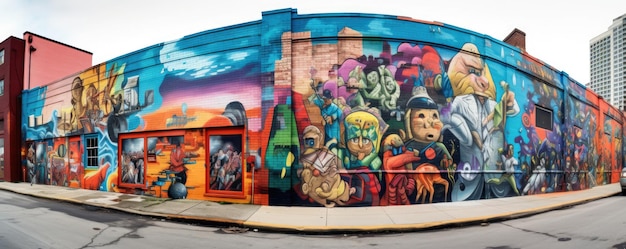This image captures a vibrant street scene featuring a uniquely designed building with a colorful mural. The building exhibits a curved, almost fishbowl-lens effect, making it appear wider in the center and narrower at the edges. Dominating the left side is a taller red building that contrasts sharply with the single-story structure adorned with a plethora of vivid colors and cartoon-like graffiti.

The mural, stretching across the building, is a kaleidoscope of hues: vivid blues, pinks, yellows, oranges, and reds. Detailed cartoons adorn the wall, including whimsical characters like a monkey in a white suit and another figure seemingly interacting with an octopus. The artwork is dynamic, with varying faces and shapes in colors like purple, yellow, red, green, and dark blue.

Towards the upper left, near the red taller building, light blue patches stand out against darker blue, evoking a castle-like appearance. Below this, green and blue shades flood the scene, mingling with the myriad cartoonish figures. Purples and reds punctuate the design, while blue windows and orange splotches add texture.

A prominent sidewalk curves alongside the building, aligning with a street marked by noticeable cracks in the bitumen. In the background to the right, a tall high-rise building looms with numerous windows, emphasizing the depth and urban setting of the scene. The overall visual is strikingly dynamic and vibrant, displaying a captivating mixture of street art and urban landscape.